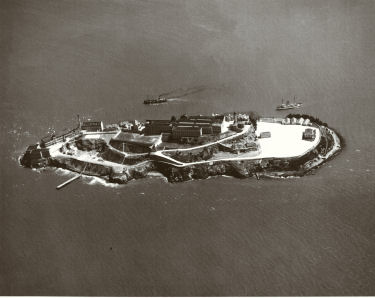This sepia-tinted black-and-white aerial photograph depicts a small island surrounded by water, diagonally positioned in the frame. The oblong-shaped island features a prominent collection of connected buildings at its center, with roads and a pier extending outward. There are visible outbuildings and a large main structure, accompanied by several low shrubs and chunks of fence lining one end of the island. Two ships are approaching or leaving the island, with one emitting smoke from its smokestack. The perimeter of the island includes a rocky cliffside, suggesting an isolated and solitary setting akin to Alcatraz. The island's sparse vegetation and pale ground contrast with the surrounding water.